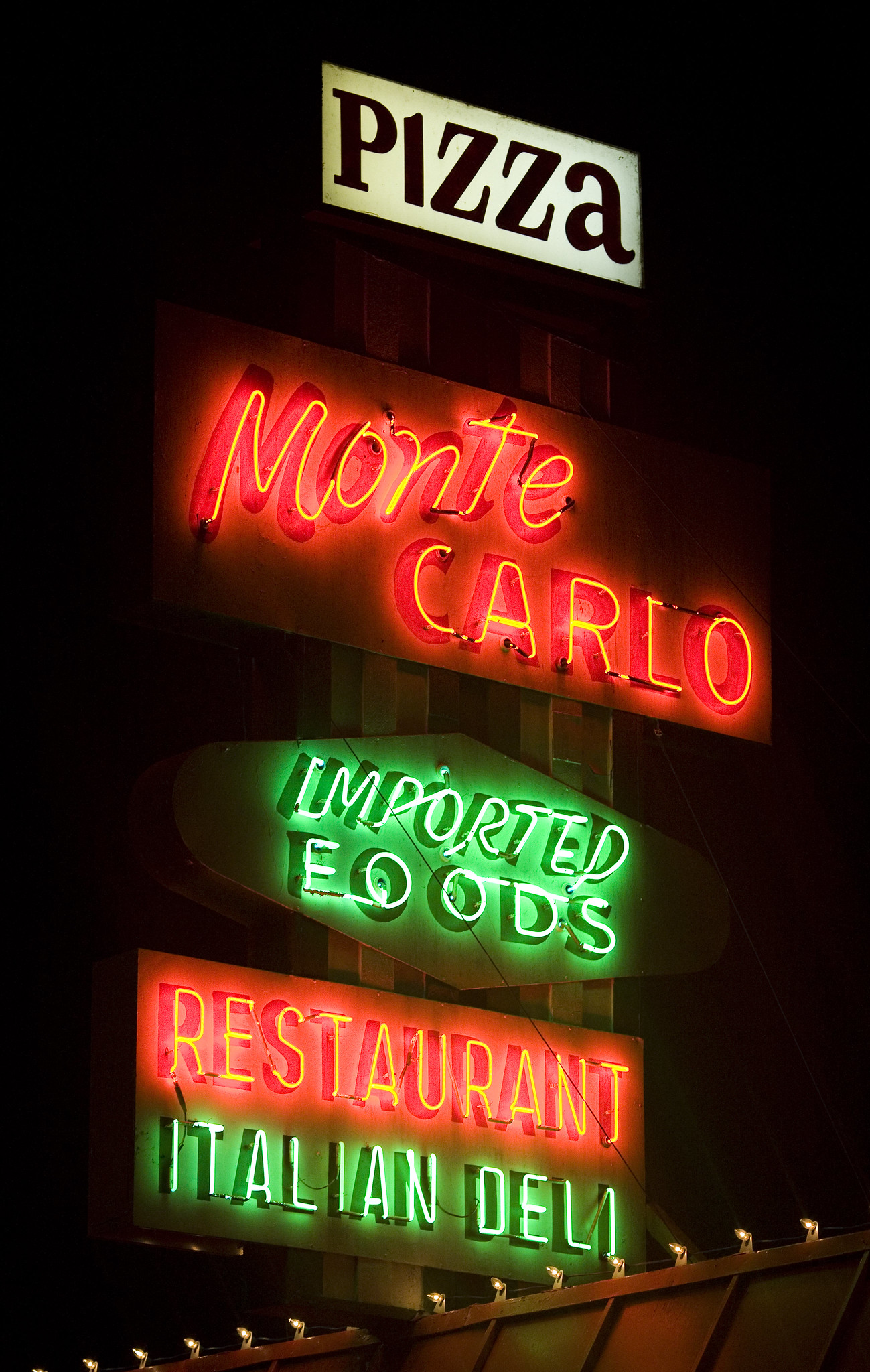The image depicts a series of vintage-style restaurant signs stacked vertically atop a building with a red tin roof, against a dark night sky. At the apex is a rectangular white sign with bold black lettering that reads "PIZZA," softly backlit to illuminate the white background. Directly beneath is a prominent neon sign that reads "MONTE CARLO" in bright yellow letters enveloped by a radiant red glow. Below it, in vibrant green neon, the sign reads "IMPORTED FOODS." The sequence concludes with the bottom-most signage, a neon-lit display that combines both red and green glows: the word "RESTAURANT" is emblazoned in yellow letters with a red glow, while "ITALIAN DELI" is presented in white letters with a green glow. Enhancing the nostalgic atmosphere, a row of small, Christmas-like lights adorns the top edge of the roof, further adding to the image's delicate nighttime charm.